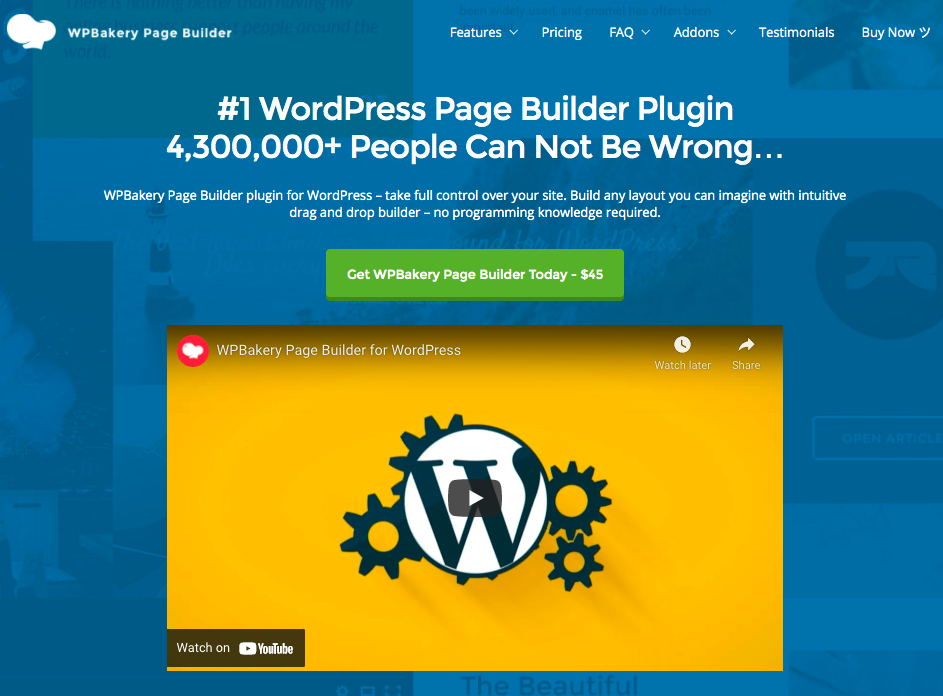The website’s interface features a visually appealing design with a blue background situated at the upper left corner. Prominently displayed is an image of a baker's hat, a classic white chef’s hat, alongside the text "WP Bakery Page Builder." Across the top are navigational columns labeled "Features," "Pricing," "FAQ," "Add-Ons," "Testimonials," and "Buy Now," all written in a clean white font.

Centrally positioned beneath these navigation links is an emphatic statement in white text: "Number one WordPress Page Builder Plugin. 4,300,000+ people cannot be wrong… WP Bakery Page Builder Plugin for WordPress. Take full control over your site. Build any layout you can imagine with Intuitive Drag and Drop Builder. No programming knowledge required."

Directly below this statement lies a prominent green call-to-action box, centered with the text: "Get WP Bakery Page Builder Today - $45."

Following the green box is a larger section with an orange background. At the top, a red circle features a white bakery hat. Next to this, the text “WP Bakery Page Builder for WordPress” is written in white font. On the left side of this section, icons indicate options to "Watch Later" or "Share." Dominating the center is a substantial white circle containing a bold black "W" accompanied by cogwheels on either side and an arrow symbol suggesting the start of a video. At the bottom, it’s noted that this video can be viewed on YouTube.